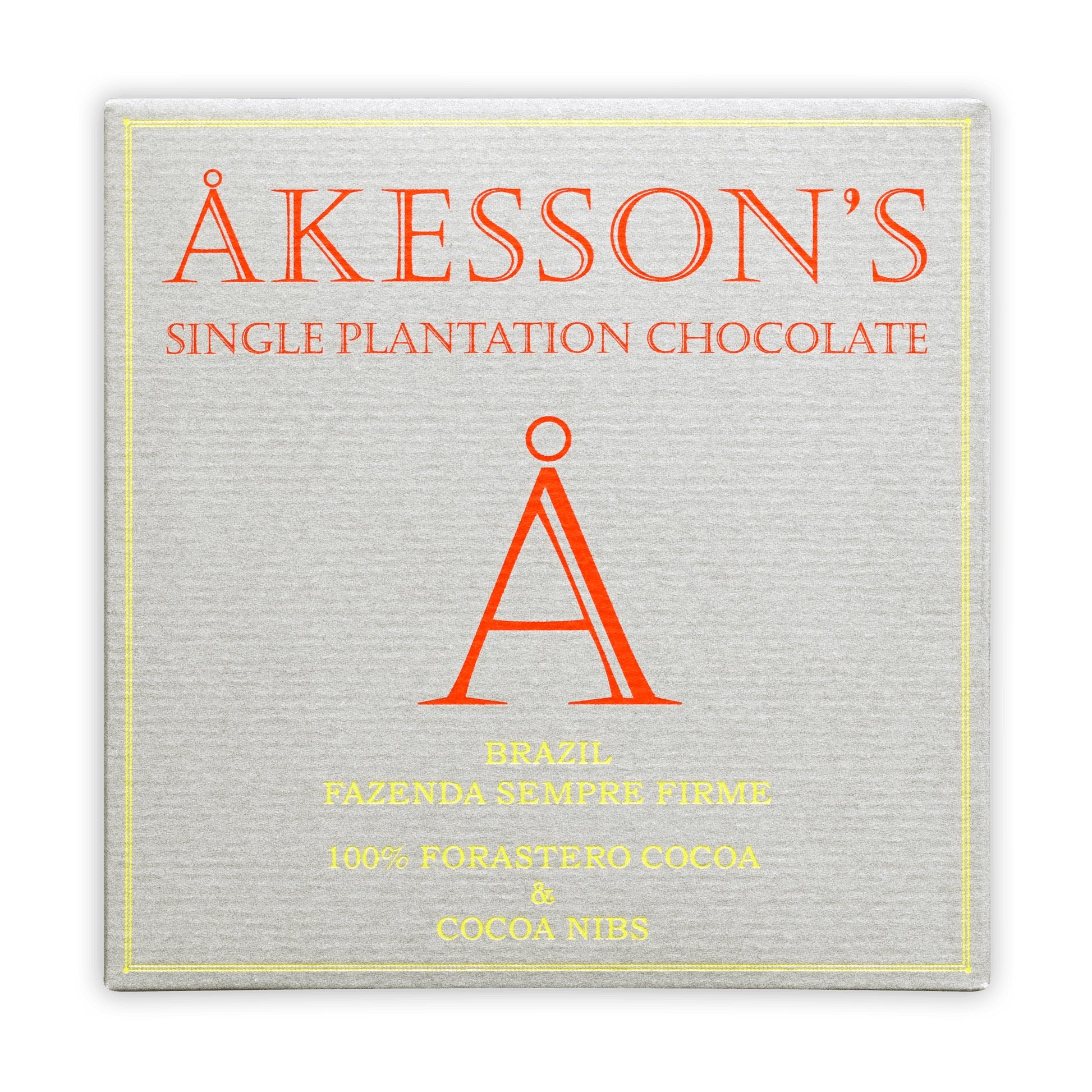This is an image of an advertisement for Akesson's Single Plantation Chocolate, prominently displayed on a grey textured square background with a thin gold border. The title "Akesson's Single Plantation Chocolate" is boldly written in red font at the top of the image. Central to the design is a large red "A" with a circle accentuating the top of it. Below this distinctive logo, the text "Brazil Fazenda Sempre Firme 100% Forastero Cocoa and Cocoa Nibs" is elegantly printed in gold, indicating the chocolate's origin and composition. The detailed grey texture of the material adds a sophisticated touch to the overall presentation.